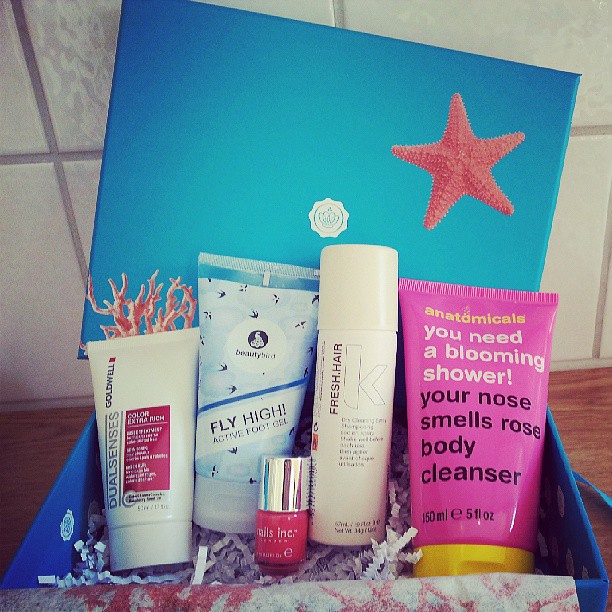The photograph depicts an open beauty or skincare subscription box placed on a wooden table with a white tile wall in the background. The box itself is blue with an image of a red starfish on the lid. Inside the box, surrounded by crinkled paper confetti, are several personal care items arranged from right to left. On the far right, there is a pink tube with a yellow cap labeled "Anatomicals: You Need a Blooming Shower, Your Nose Smells Rose Body Cleanser." Next to it is a white bottle labeled "Fresh Hair," likely a dry shampoo. Moving left, there is a smaller canister which appears to say "Nails Inc" and is reddish at the bottom, transitioning to a metallic color at the top. Further left is a baby blue tube labeled "Fly High Active Foot Gel." On the far left, there is another white tube with text that's partly unreadable, possibly "DualSense Color Extension High." The interior of the box and the lid also feature pink coral and a pink starfish, along with a white insignia in the center, which may represent the brand's logo.